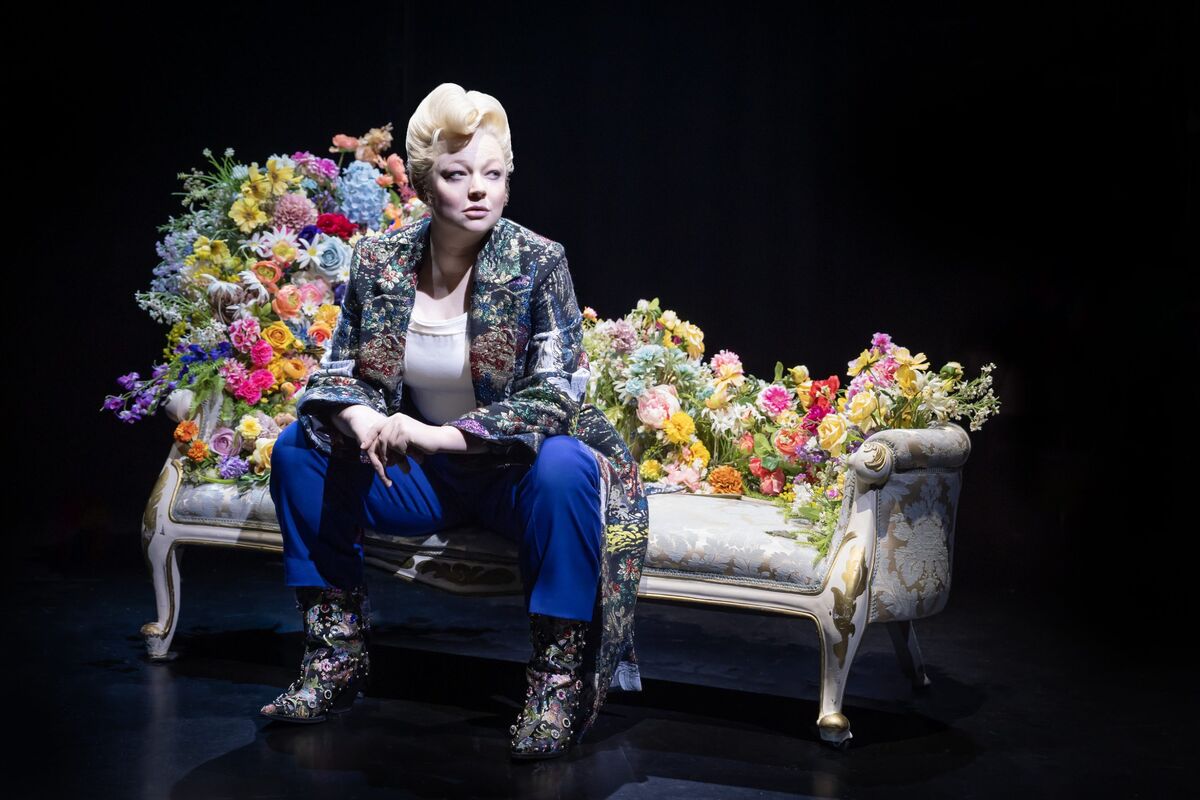This photograph captures a woman seated on a lavish, Victorian-style bench adorned with a massive array of multicolored flowers along its backrest, creating a dramatic and ornate backdrop. The flowers cover the upper and side portions of the bench so densely that it appears one couldn’t comfortably recline against them. The stage is dark, accentuating the spotlight on the woman and the vibrantly decorated bench.

The woman, likely in her 30s or 40s, has short blonde hair pulled back. She dons a striking multicolored long coat featuring floral designs, complementing her white long-sleeve sweater underneath. Her attire also includes blue slacks and distinct, fanciful boots decorated with images of roses and various ornaments, which mirror the floral pattern on her jacket. She sits in a confident pose, legs wide apart with elbows resting on her knees, capturing both her robust demeanor and the intricate, flower-loaded setting. This detailed interplay between her elaborate clothing and the floral embellishments of the bench enhances the theatrical ambiance of the scene.